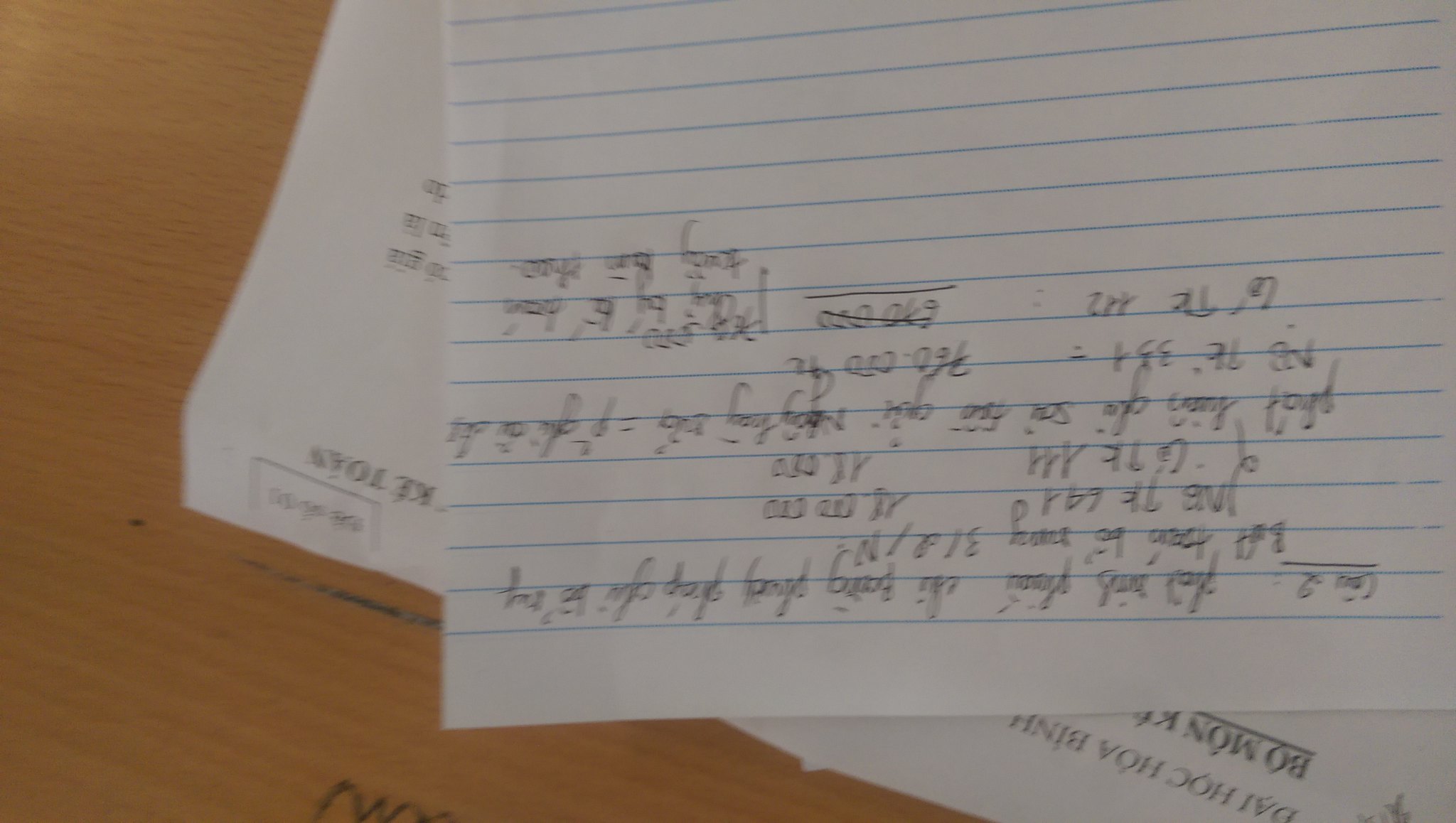The image depicts two pieces of paper placed on a faux wood desk with an oak finish. The photograph has been taken upside down, presenting a challenge in interpreting the content, which appears to be written in a Southeast Asian language, possibly Thai or Vietnamese. The bottom page is a black-and-white Xerox copy, featuring all-caps text in a serif font, with a combination of bold and regular type. The top page is neatly placed college-ruled notebook paper, characterized by its blue lines and smooth edges, without any visible holes or ragged marks. The handwriting on this page is exceptionally neat and consistent, showing a slight leftward slant. The text comprises both uppercase and lowercase letters, accompanied by some unfamiliar characters.